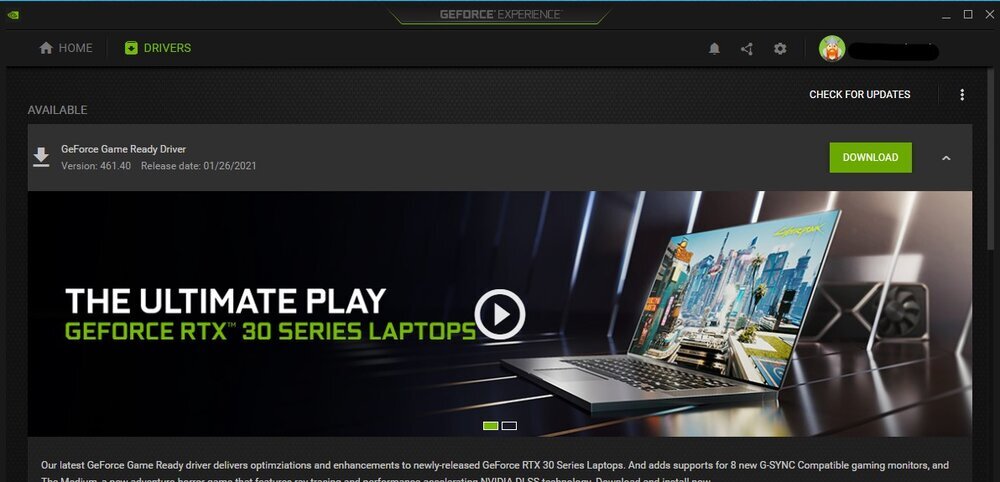The screenshot is from the Nvidia GeForce Experience software, showcasing the driver update section. At the top center, the title "GeForce Experience" is prominently displayed. In the upper left corner, the Nvidia logo is visible. Directly below the logo is a horizontal navigation bar. On the left side of this bar are the "Home" and "Drivers" buttons, with the "Drivers" button highlighted in green, indicating it is the currently selected option.

In the main content area below the navigation bar, the word "Available" appears in gray. Beneath this, the text "GeForce Game Ready Driver" is shown, followed by the version number "461.40." Additionally, the release date "January 26th, 2021" is noted. To the right of this information is a prominently placed "Download" button.